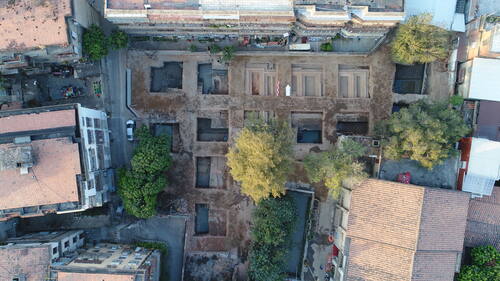This aerial, horizontal landscape-oriented photograph captures a top-down view of a residential area surrounded by buildings with visible rooftops on the left, top, right, and lower right edges. At the center, there is what appears to be a large concrete courtyard with a series of recessed plots, hinting at a lower level beneath it, reminiscent of an archaeological site. The courtyard is framed by various treetops—dark green, brighter green, and yellow hues—providing a vibrant contrast against the urban structures. Specifically, a prominent yellow treetop is centrally located, with other treetops positioned towards the left corner and upper right corner. The scene also includes parked cars, notably a white one on the left side near a street intersecting the area.